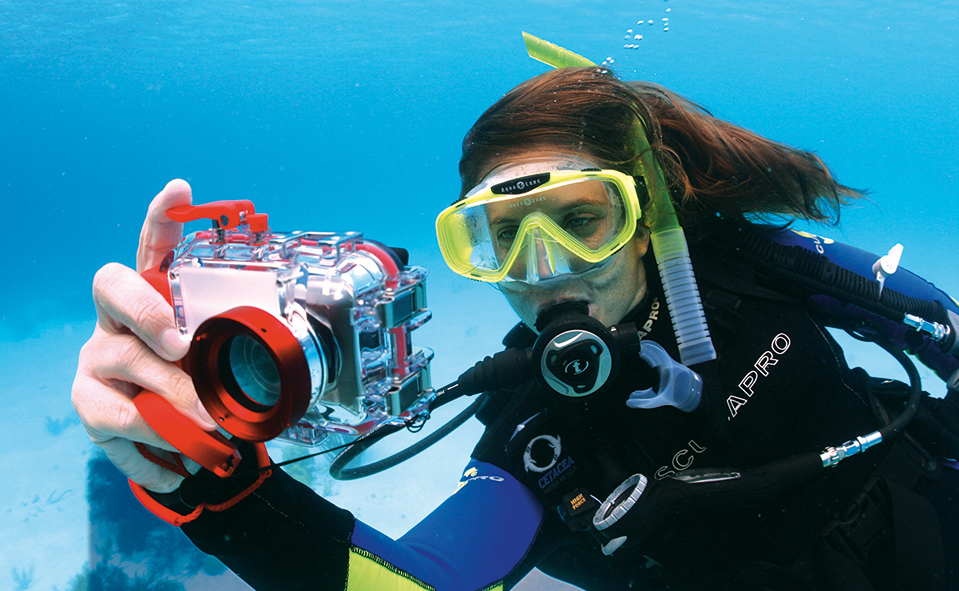An underwater scene captures a woman with long, dark, flowing hair wearing a black wetsuit that reads "Aperol" and "Cetacea." She has on clear, 3D goggles framed in yellow and a matching snorkel. Her face is partially obscured by a mouthpiece connected to her oxygen tank, with tiny bubbles rising from it. The woman is positioned diagonally from the bottom right to the center of the image, her right hand outstretched towards the bottom left corner, holding a white and red underwater camera, poised to take a picture of an unseen subject. The background is a serene, clear blue with subtle hints of oceanic colors such as see-through yellow, bright shiny red, orange, clear blue, yellow, and beige, encapsulating the essence of an underwater environment. Her hands appear slightly crinkled from prolonged exposure to the water.